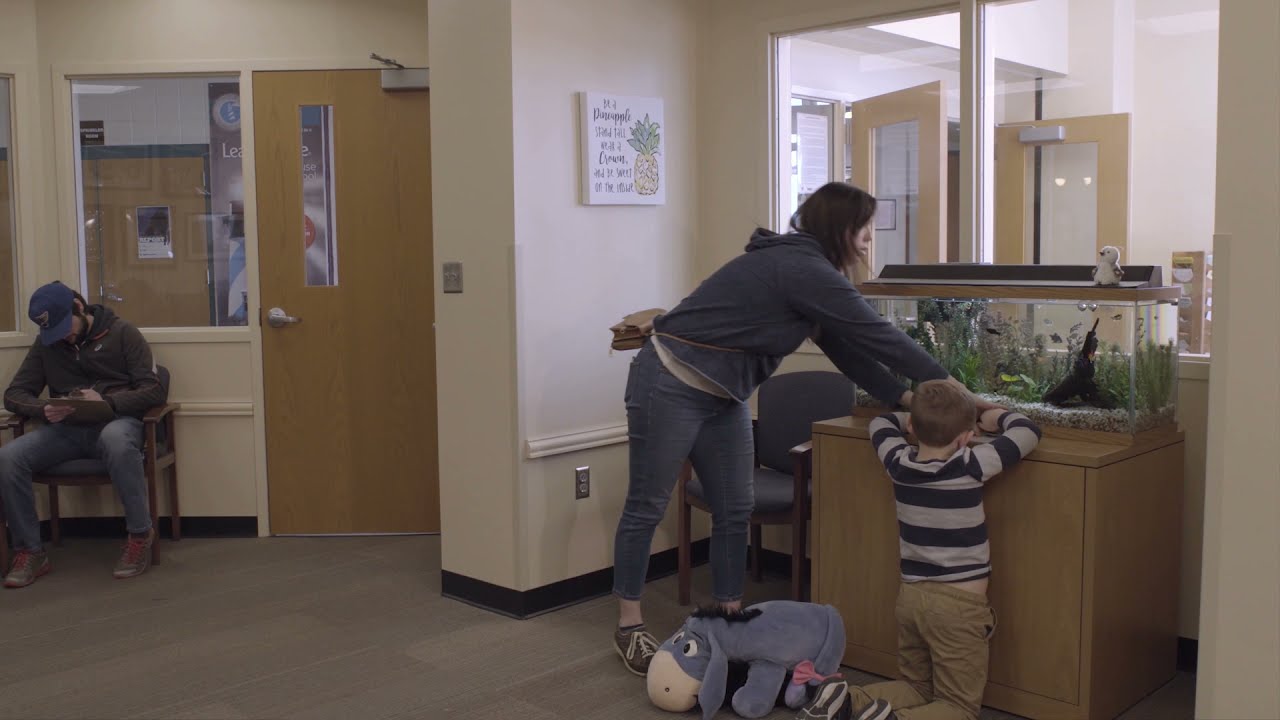This image captures a typical scene inside a doctor's office waiting room, characterized by its beige and brown hues. At the center of the room, a young boy, approximately seven years old, dressed in a blue and white striped shirt and brown khakis, is intently observing a fish tank placed on a cabinet. Beside him sits a blue Eeyore stuffed animal. His mother, clad in blue jeans and a hoodie, leans over to join him in watching the fish, possibly explaining the details to him. To their left, a man in a hat, jeans, and a jacket sits near the door, engrossed in filling out a clipboard. The room features multiple doors and windows, including a large window that opens to the hallway outside. On the wall is a picture featuring a pineapple, while in front of the doors is a solitary blue chair. The scene is completed by a gray floor, typical of waiting rooms in medical facilities.